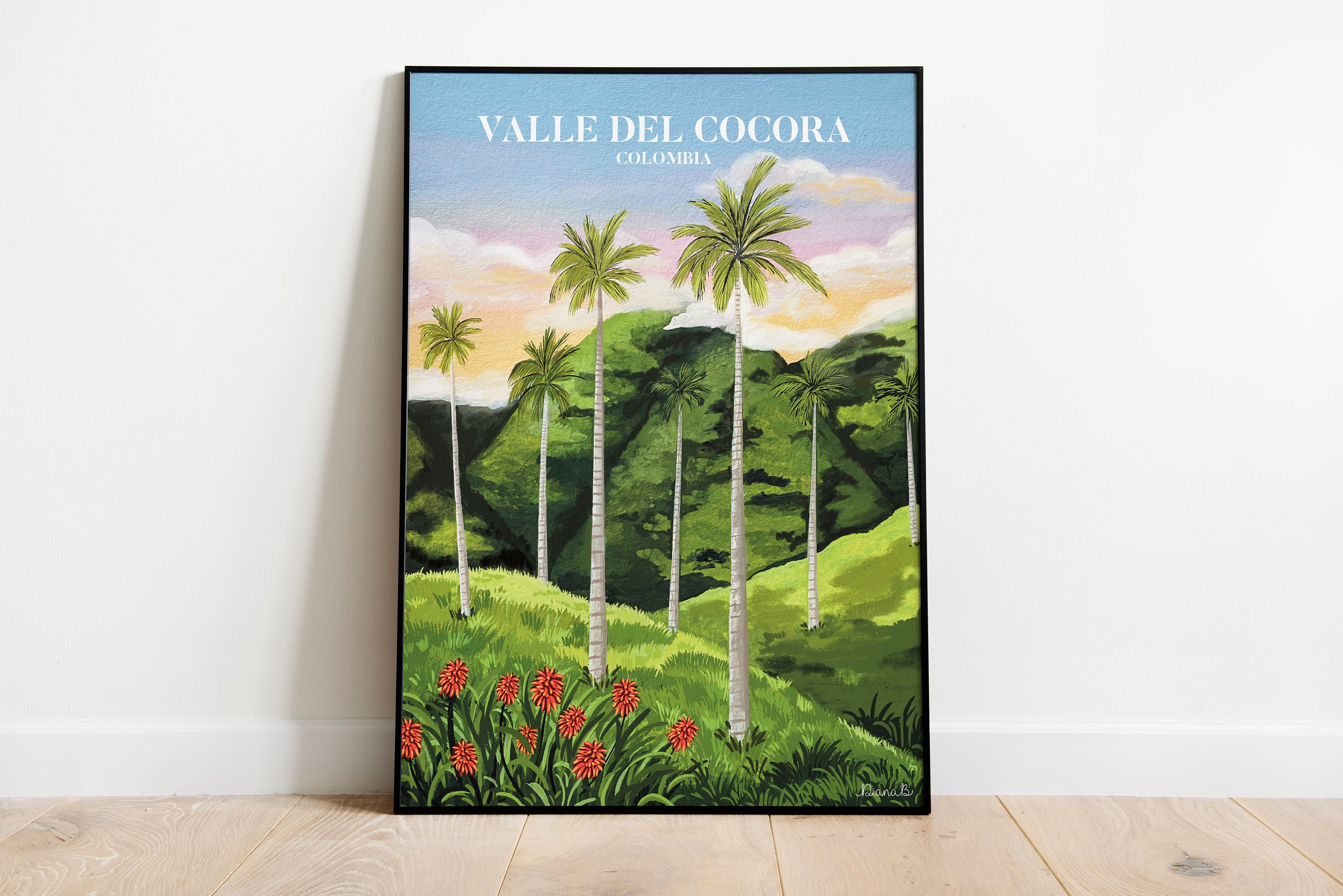The image features a framed artistic poster propped against a white wall atop a traditional wooden floor, bordered by a thin white skirting board. The poster is enclosed in a thin black frame and depicts a vibrant natural scene titled "Valle del Cocora, Colombia" in white text at the top. The artwork illustrates a lush, green landscape with several tall, slender palm trees featuring clusters of leaves at their tops, set against a backdrop of rolling hills with wide and steep slopes. Some hills are dome-shaped and display varying shades of green. Additionally, the foreground is adorned with red flowers in the bottom left corner. Above, blue skies are scattered with wispy pink and yellowish clouds, giving the impression of either a sunrise or sunset. This image likely serves as a product photo, showcasing what the framed poster looks like in a home setting.